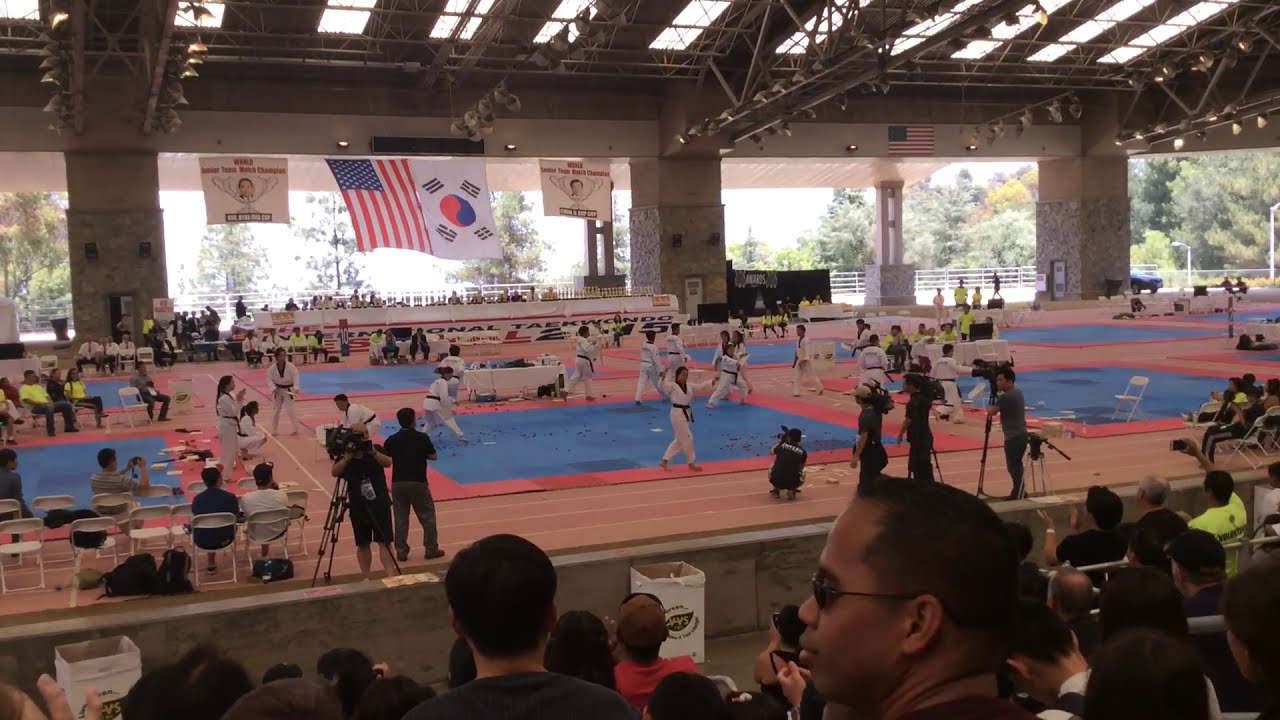This detailed photograph captures a large national Taekwondo tournament taking place in an indoor stadium. The scene is bustling with activity, featuring more than a dozen participants practicing their Taekwondo moves on mats that are primarily blue with red outlines, laid out in a spacious area on the stadium floor, which is light brown. Spectators fill the stands, attentively watching the tournament unfold. The participants are dressed in traditional white uniforms with colored belts indicating their rank. Numerous coaches and judges are present, seated on the sidelines, contributing to the structured environment of the competition.

The photograph also captures the presence of various media personnel, equipped with cameras and video equipment, indicating that the event is well-documented. The atmosphere is enriched by the display of international flags, notably those of the USA and South Korea, hanging prominently in the middle of the stadium. The open walls of the stadium provide a glimpse of the outside area, showcasing trees and offering a sense of openness to the otherwise energetic indoor setting. Additionally, a banner in the background confirms the nature of the event, reading "Invitational Taekwondo," which further underscores the significance of this national-level competition.